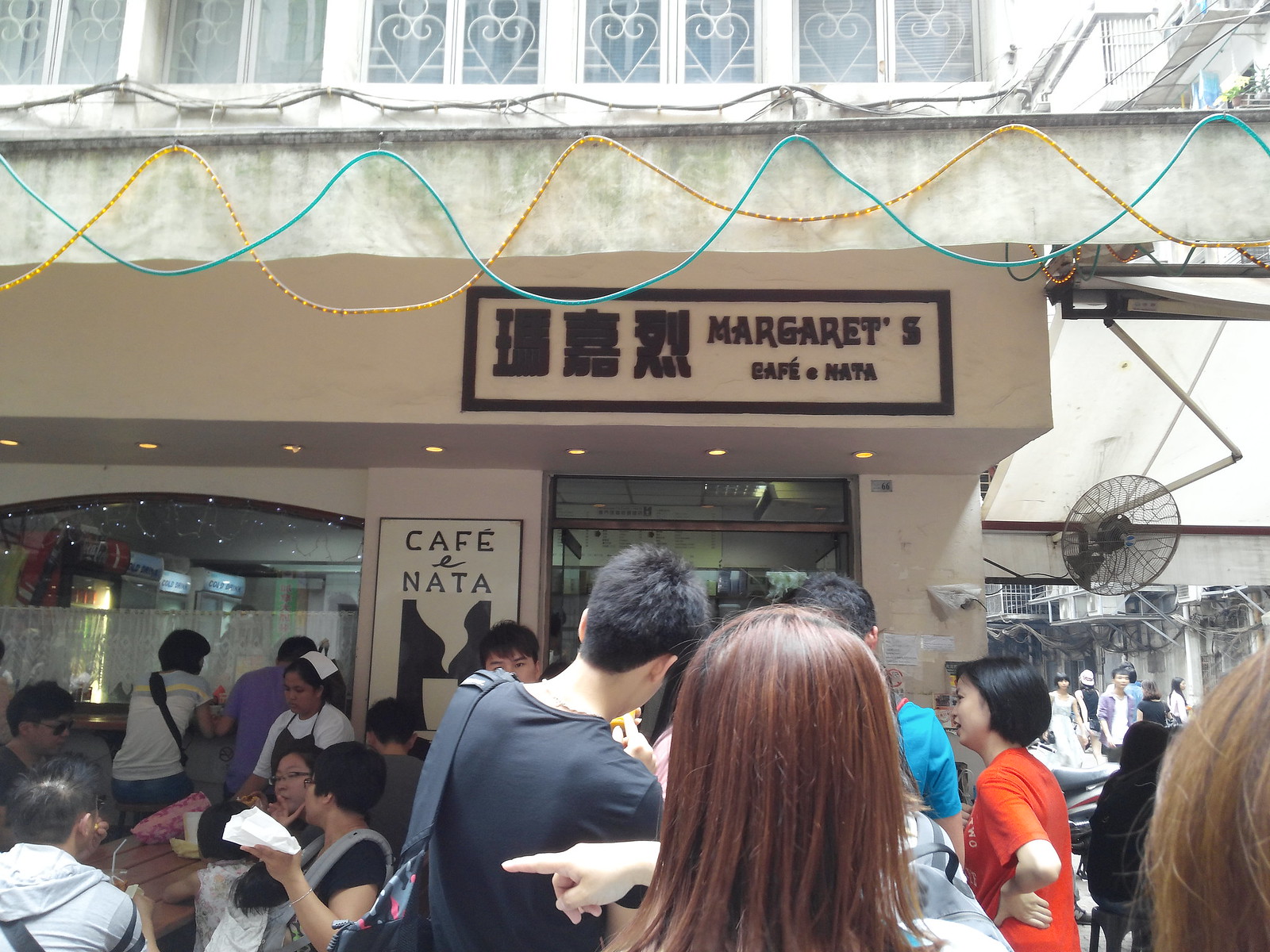The image depicts a bustling outdoor scene of Margaret's Cafe Nada, a popular cafe with a light brown, brownish-gray facade adorned with Japanese lettering and signage that reads both "Margaret's Cafe" and "Cafe Nata." The cafe serves as the backdrop, featuring large entryways and a row of windows above which string lights—yellow and blue—are hung, suggesting the cafe transforms beautifully at night. A large outdoor fan is mounted on the wall to the right. The area is crowded with both seated and standing patrons, some of whom appear to be waiting in line, while others look through the windows, indicating the cafe's high popularity.